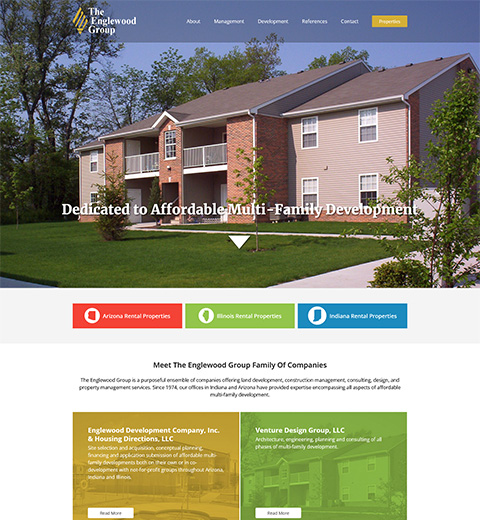The image depicts a website, slightly taller than it is wide, featuring a prominent banner across the top half. This banner showcases an external view from a street corner, highlighting a two-story house situated on a corner lot. The house is characterized by three brick pillars in the front and two white balconies on the second floor. These balconies span between the pillars and are complemented by two porches on the first floor, though the interiors of the porches are not visible. The exterior of the house is a tan color, and it features four windows arranged in two equal sections on each side.

Overlaying the image, there is text at the bottom of the banner that reads, "Dedicated to affordable multifamily development." Above the banner, the website's semi-transparent menu bar is visible. It includes the title "The Englewood Group," accompanied by a logo on the left, which is a yellow diamond made of diagonal stripes pointing towards the one o’clock direction. The menu bar consists of around five options and features a yellow "Register" button on the right.

Below the main banner, the text "Meet the Englewood Group family of companies" is displayed, followed by two colorful sections, each containing a paragraph of text and providing further information about the group.